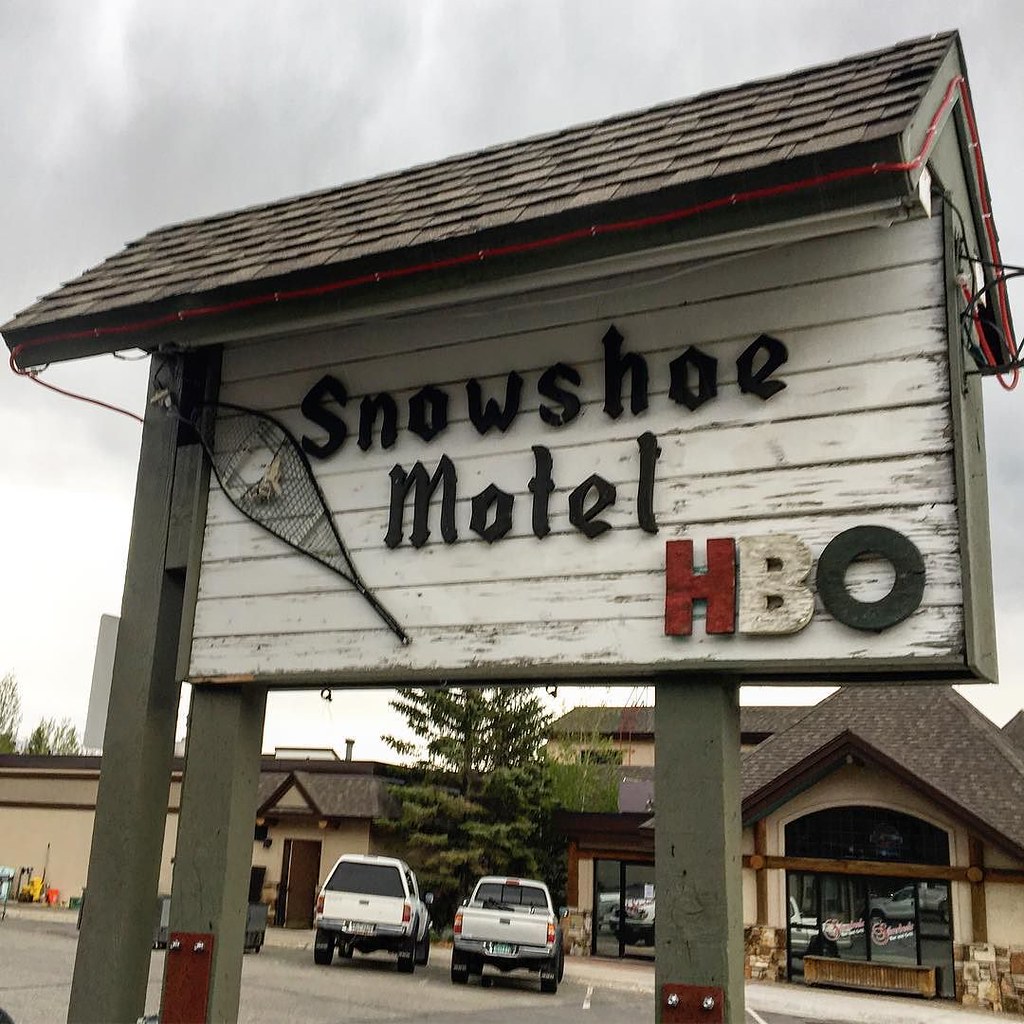The image captures the front of the Snowshoe Motel, showcasing a distinctive white wooden sign with a V-shaped roof and supported by green posts. Prominent in the foreground, the sign features "Snowshoe Motel" in black lettering alongside a black ski foot racket illustration, while promoting HBO with red, white, and black text. The sign is adorned with wires, indicating it lights up at night. Behind the sign, the beige motel building with a brown roof is visible, complete with multiple windows leading into the facility. Two white trucks are parked in the lot, along with cleaning supplies and boxes positioned outside. Red and white lettering is faintly seen on the door, enhancing the detailed, yet bustling facade of this roadside lodging.